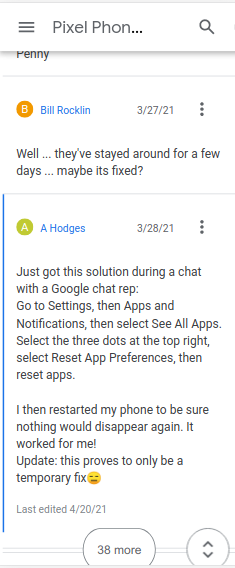The image depicts a screenshot of a search performed on a Pixel phone. In the top left corner, the search term appears to be cut off but indicates "words pixel phone." On the right, there's a magnifying glass icon, likely for initiating new searches. Below this, two comments are shown with details:

1. The first comment is by Bill Rocklin, dated 3-27-21. His comment reads, "Well... they stayed around for a few days... maybe it's fixed."

2. The second comment is by A Hodges, indicated by a green initial circle, dated 3-28-21. This comment provides a step-by-step solution received during a chat with a Google representative: "just got the solution during a chat with a Google chat rep. Go to settings, then apps and notification, and select see all apps. Select the three dots at the top right, and then select reset app preference, then reset the apps. I then restarted my phone to make sure nothing would disappear again. And then wait for main update. This proves to only be a temporary fix."

Additionally, the initial of Bill Rocklin is shown in an orange circle. The image seems to document a troubleshooting thread related to a recurring issue with the Pixel phone.